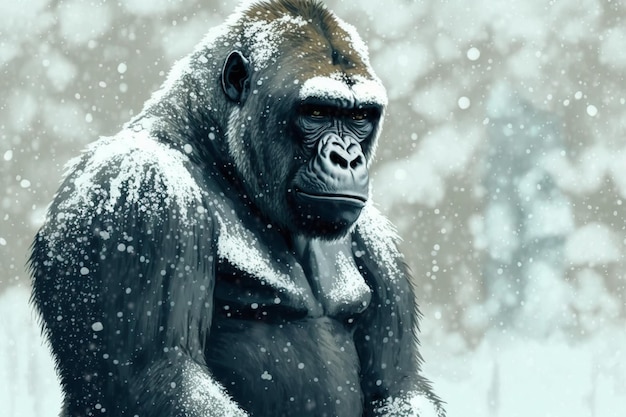This image captures a formidable gorilla in a snowy landscape, evoking the iconic presence of King Kong. The gorilla's dark, muscular upper body is prominently displayed as it stands tall, revealing powerful arms and an imposing chest dusted with snow. His intense gaze is directed straight ahead, with a slightly downward tilt of his head, showcasing his black face adorned with wrinkles and snow-tipped brow bones. Snowflakes continue to fall around him, accumulating on his shoulders, head, and chest, indicating he has been sitting in this spot for some time. Despite the cold setting, the gorilla appears unfazed, emitting a sense of strength and composure with a smug, almost angry expression. The blurred background, with faint traces of snow-covered trees, further accentuates the striking image of this majestic animal in a wintry environment.